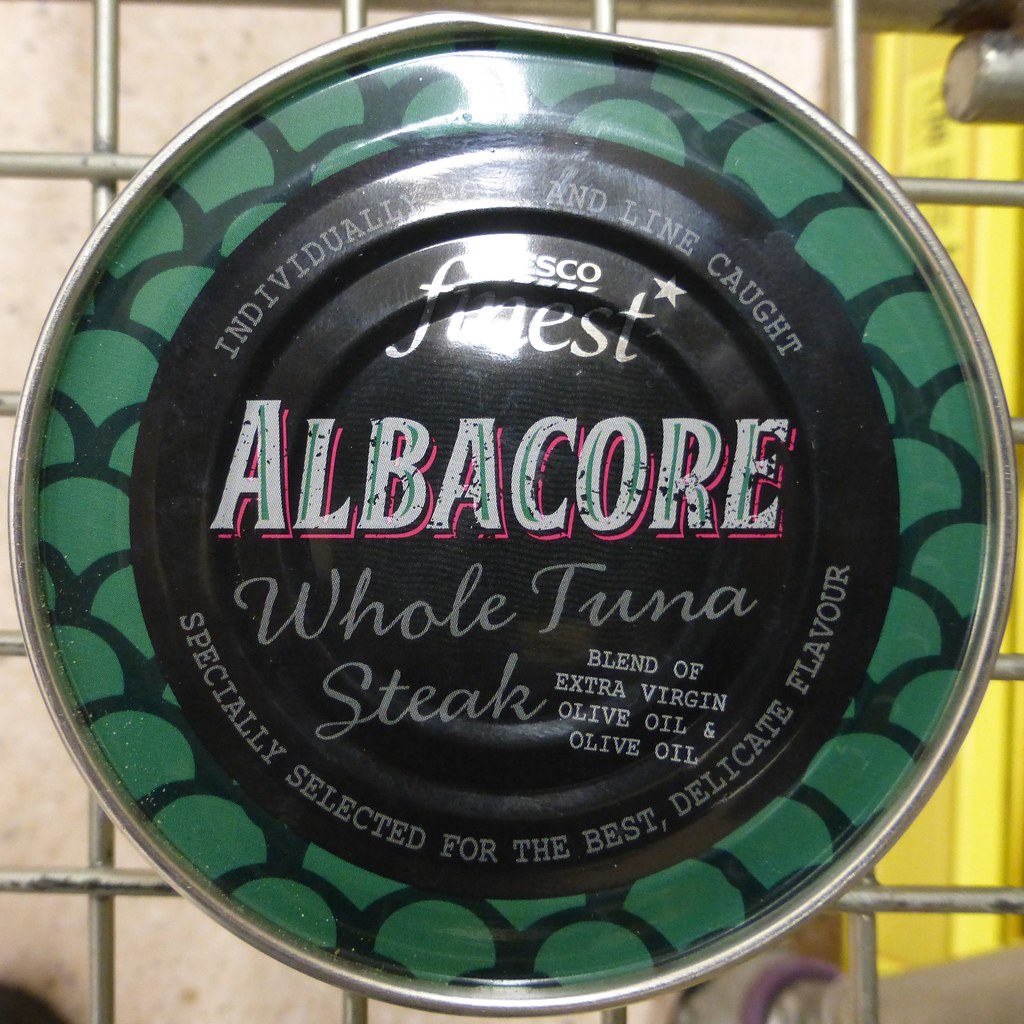In the image, we see an overhead view of a round tuna can sitting on a metal grate, likely a shopping cart, with the silver of the cart and floor visible underneath. The can's top is somewhat reflective, making the text a bit difficult to read due to the lighting. The outer edge of the can has a green design resembling a spider web or a turtle shell. Inside this green border is a black circle containing various texts in gray and white lettering. The text reads as follows: "Individually and line caught," followed by "Casco Finest," and below that, "Albacore Whole Tuna Steak." It also mentions "Blend of extra virgin olive oil and olive oil" in white text, and further down, it says, "Specially selected for the best delicate flavor."